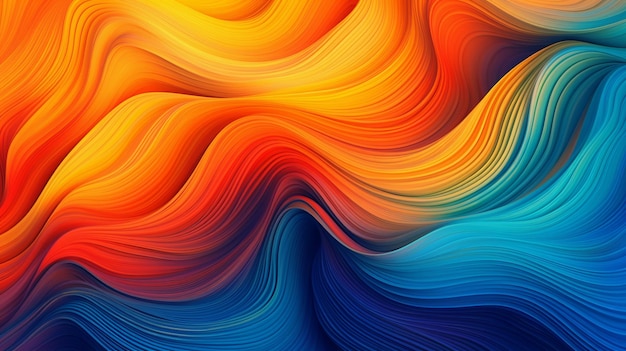This rectangular piece of art features vibrant, swirling layers of color that evoke the fluid movement of hair or fabric. The composition is divided with the top three-fourths dominated by an orangish-yellow blend while the bottom quarter is immersed in varying shades of blue. Starting from the middle left and stretching to the right, the colors transition from deep reds to bright oranges and golden yellows, creating a sense of flowing movement. The deepest reds dominate the circular middle section, with the colors lightening as they expand outward. The bottom section transitions from dark blues and purples on the left to robin's egg blue towards the middle right. Some hints of green appear where the blue meets yellow in the right middle section, adding subtle complexity to the ribbony, flowing forms. The whole image exudes an abstract, dynamic energy, with colors scrunching up more towards the lower left and flowing outward more expansively towards the top, middle, and far right.